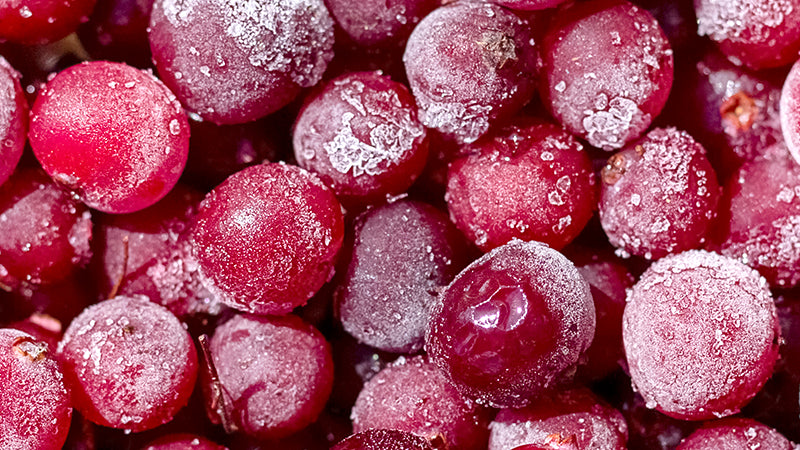The image depicts a close-up of a cluster of reddish-purple round fruits, likely frozen grapes or possibly cherries or cranberries. These fruits exhibit varying shapes and sizes, with some appearing slightly deformed or indented, indicating that not all of them are in perfect condition. A significant number of the fruits are covered in a white, frost-like substance, suggesting they have been stored at very cold temperatures, possibly in a freezer. The frost forms tiny droplets or splotches on the surface of the fruits, highlighting their juicy and glossy texture under a high light source. The fruits are closely packed together, touching each other, and the background remains indeterminate as the focus is sharply on the fruits themselves, creating a vivid contrast with their ruby or burgundy hues.